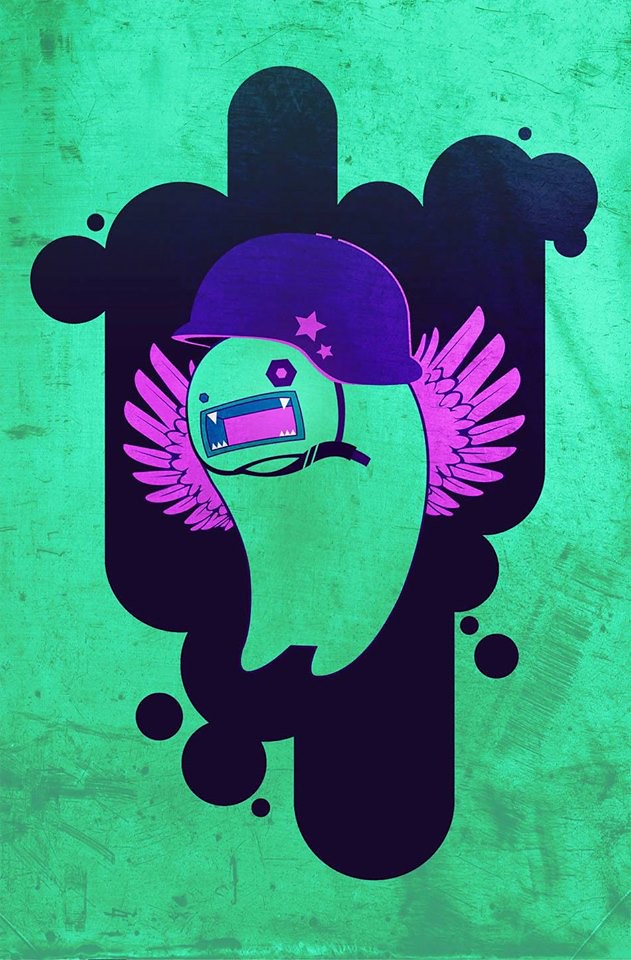The image presents a highly stylized, vibrant green background marked by splotchy, weathered textures. Central to the composition is an animated green creature, resembling a fish with a raindrop-shaped body and two appendages at the bottom. Perched on its head is a distinctive, navy blue army general's helmet adorned with two pink stars. The creature's face is dominated by a wide, rectangular mouth filled with jagged teeth—two sharp incisors at the top, and six fangs on the bottom. A smaller rectangle inside the mouth indicates its gullet, and the tongue is a noticeable pink rectangle. The creature has asymmetrical eyes: one is a simple dot, while the other is a red circle with a hexagonal pattern around it. Elegantly extending from each side of its body are two pink wings, adding a whimsical touch. The green figure stands out against an oddly shaped black background, composed of several interconnected oval shapes that seem to form a tall, squished structure, decorated with circular elements. This black area enhances the vividness of the green background, making the cartoon-like character the focal point of the image.